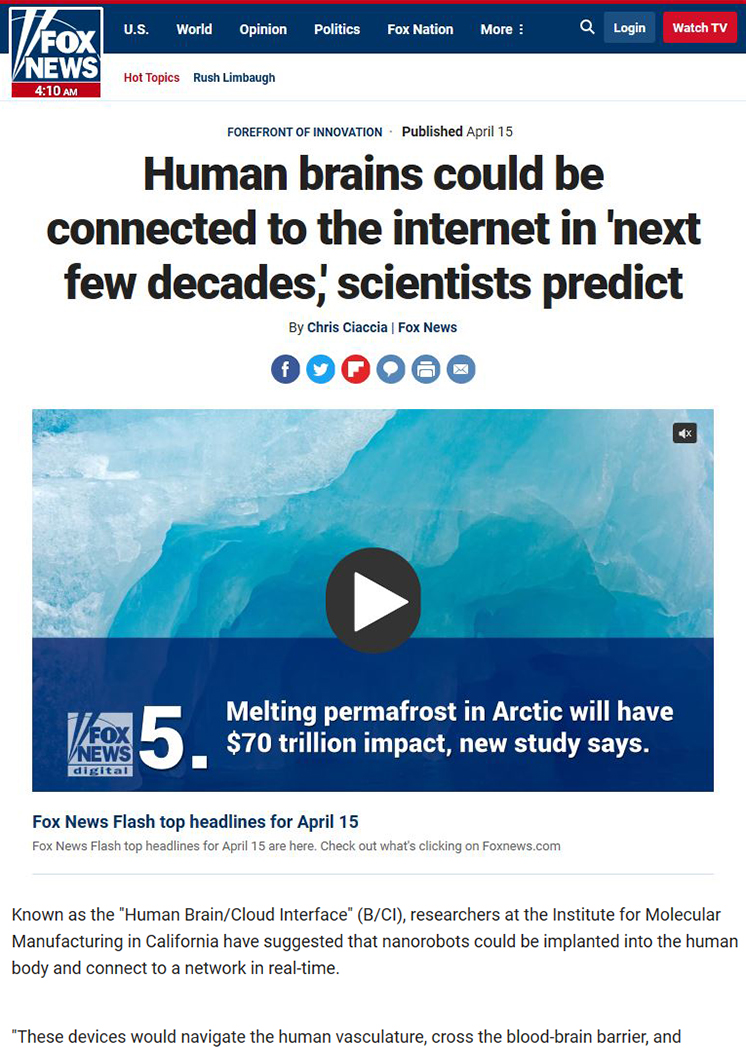On this image is the Fox News website. The top left corner prominently features the "Fox News" logo in white against a blue background. Just below the logo, a red box displays the time as "14 AM." Across the top of the page, several navigation tabs are listed in white text on a blue background: "US," "World," "Opinion," "Politics," "Fox Nation," "More," and a search button. On the top right, there are "Login" and "Watch TV" buttons; the "Watch TV" button is red, and the "Login" button is blue.

On the left side, it says "Hot Topics: Rush, Limbo." Below that is a headline reading "Forefront of Innovation," published on April 15, discussing the possibility that human brains could be connected to the internet in the next few decades, as predicted by scientists. The byline attributes the article to Chris Siasia from Fox News. Beneath the headline are social media and interaction icons for Facebook, Twitter, Messaging, Email, and Print.

Further down, there's a video with a grey and white play button. The background of the video shows an icy landscape with blue water and white ice. The video headline at the bottom reads: "Fox News Digital 5: Melting permafrost in Arctic will have $70 trillion impact, new study says." Below the video, the text reads: "Fox News Flash Top Headlines for April 15. Fox News Flash Top Headlines for April 15 are here; check out what's clicking on foxnews.com."

At the very bottom, more detailed text discusses the "human brain/cloud interface" proposed by researchers at the Institute of Molecular Manufacturing in California. It suggests that this technology could be implanted into the human brain and connect to a network in real time, navigating the human vasculature and crossing the blood-brain barrier.

The overall background of the webpage is white.